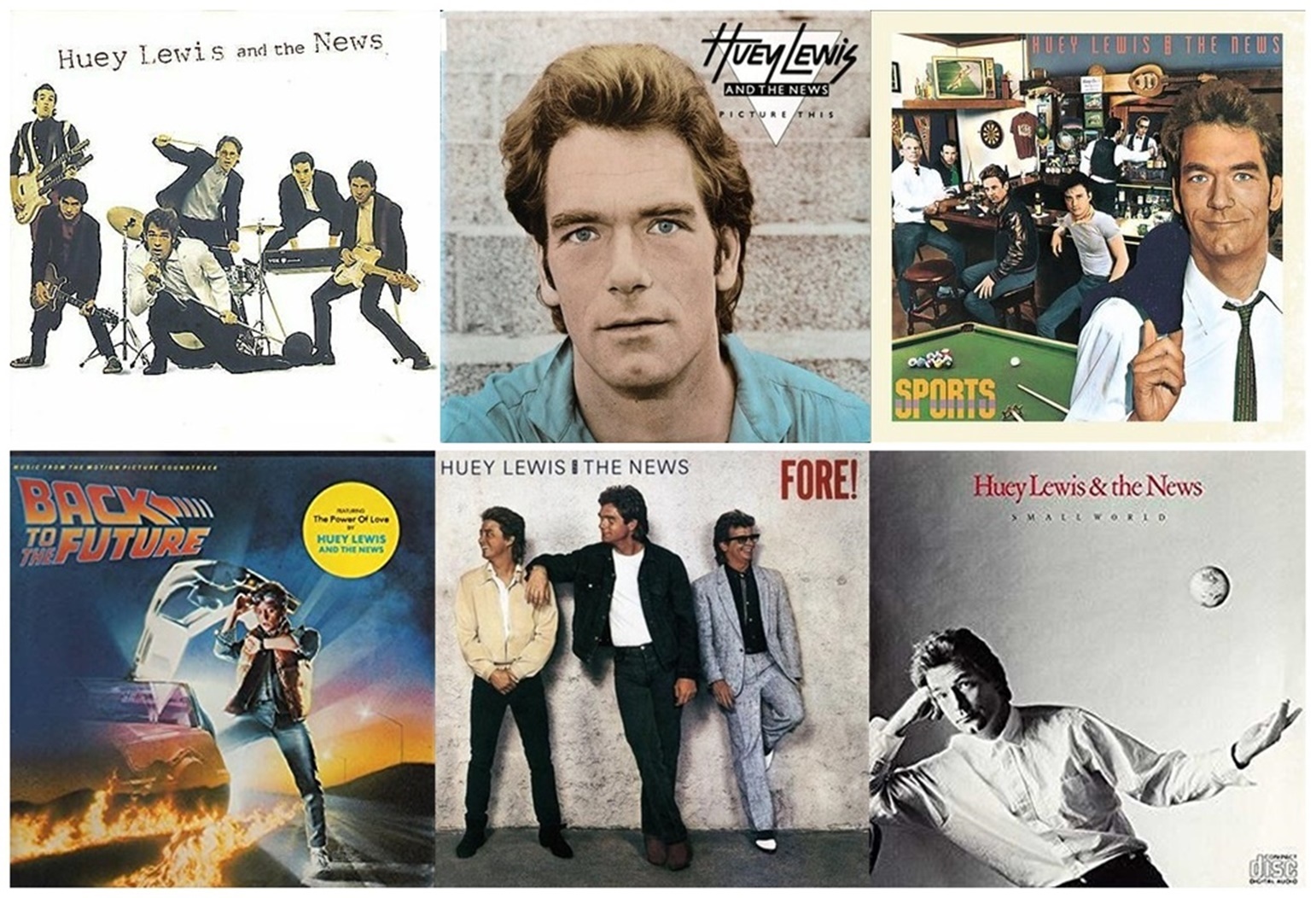The image displays six vinyl album covers from the 1980s, all featuring Huey Lewis and the News. In the top left, we see the band members playing drums and guitars while dressed in dark suits with white shirts. Next to it, there's a cover with a close-up of Huey Lewis' face, showcasing his tousled light brown hair and a blue shirt. To the right of this, another cover depicts the band in a bar setting, with Huey Lewis in a white shirt and tie, and other band members seated on bar stools near a billiards table. In the bottom row, the covers continue with varying styles: the notable one on the right is the soundtrack for the 1985 movie Back to the Future, featuring Michael J. Fox on the cover. Huey Lewis and the News created two iconic tracks for the film, with "Back in Time" being a favorite. Among the other albums is "Sports," another favorite, located in the upper right. The collection showcases the visual and musical diversity of Huey Lewis and the News during their peak in the 1980s.